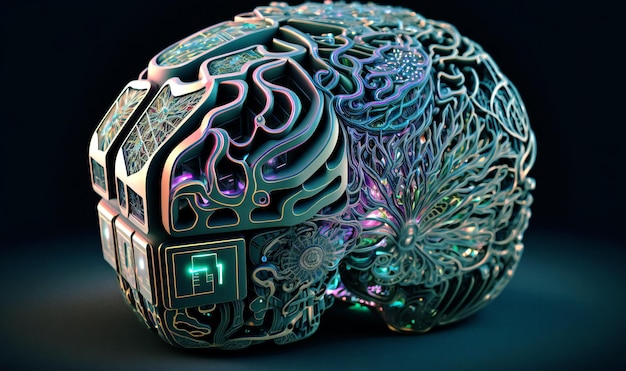This computer-generated artwork presents a vibrant and iridescent depiction of a mechanical human brain against a dark blue, almost teal backdrop. The brain-like structure is intricately detailed with a metallic finish, showcasing a stunning array of colors including greens, golds, purples, pinks, and blues. These vivid hues give the piece a holographic effect and an otherworldly shimmer. 

Technological elements, such as computer chips and wiring, are seamlessly integrated within the brain’s folds. The left side features intricate green wiring with purple outlines, weaving through in a pattern reminiscent of neural pathways. A prominent square microchip on the front glows green, adding to the artwork's luminous quality. The entire piece draws attention with its bright pink internal glow and iridescent surface, creating a captivating blend of organic brain structure and advanced technology.